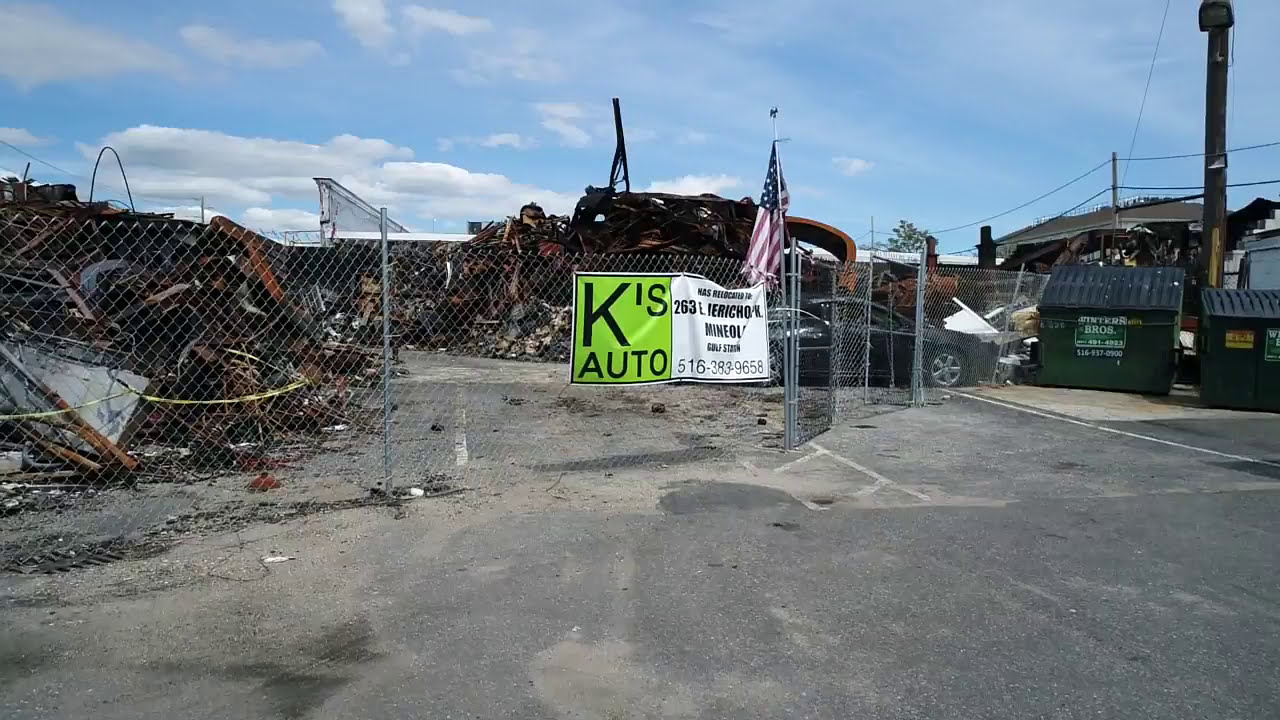The photograph captures a detailed scene at the entrance of Kays Auto wrecking yard, taken from street level in a parking lot. Dominating the middle of the image is a chain-link cyclone gate with a white sign that reads "Kays Auto, 263 East Jericho Mineal," accompanied by the phone number "516-383-9658." Adjacent to the sign, an American flag is prominently displayed, extending over the fence. On the right side of the gate, two large green dumpsters labelled "something bros" are situated, one slightly smaller than the other.

In the background, behind the fence, the yard is filled with heaps of scrap metal, including mounds of rusty pieces and a pile of crushed cars. A black car, seemingly undamaged, is parked directly behind the American flag. Further back within the yard, a white building, possibly a house, stands. The overall style of the photograph is realistic, captured in color and landscape orientation, vividly portraying the gritty atmosphere of the junkyard.